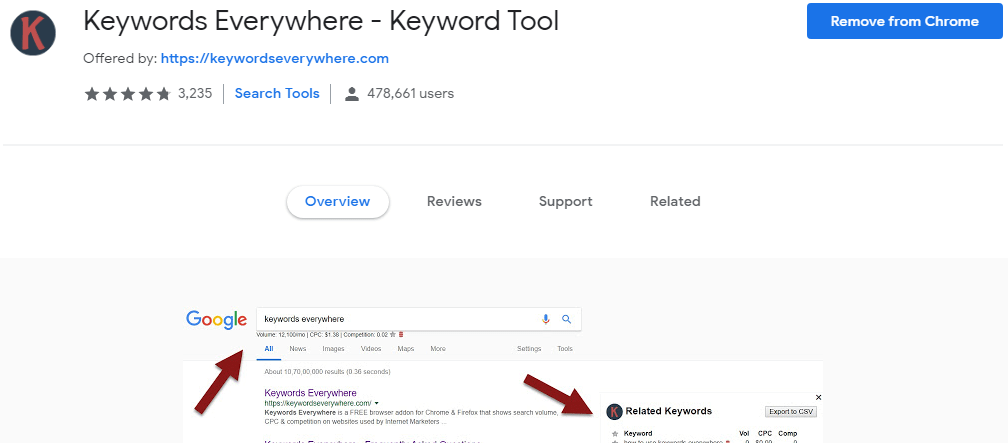The image showcases an extension for Chrome, prominently featuring the Keywords Everywhere tool. On the left side, there is a recognizable red 'K' inside a black circle. Adjacent to this emblem, the text reads "Keywords Everywhere," followed by a dash and "Keyword Tool." Below this header, it mentions that the extension is "Offered by keywordseverywhere.com." 

To the right, within a blue rectangular button, it states "Remove from Chrome." Directly beside this button, there are five gray stars and the number "3,235," indicating user reviews. Following this, a small vertical line separates the review count from the category "Search Tools," and another vertical line before noting "478,661 users."

Further down, the image highlights a navigation bar with "Overview" encircled in blue, along with tabs labeled "Reviews," "Support," and "Related."

At the bottom left corner, the Google brand logo is visible, lending authenticity. In the center of the image, inside a search bar, the term "Keywords Everywhere" is entered. An arrow points upwards to this text, while another arrow points down to a section called "Related Keywords," which again features the red 'K' inside the black circle. There is also small, unreadable text beneath "Keywords Everywhere."